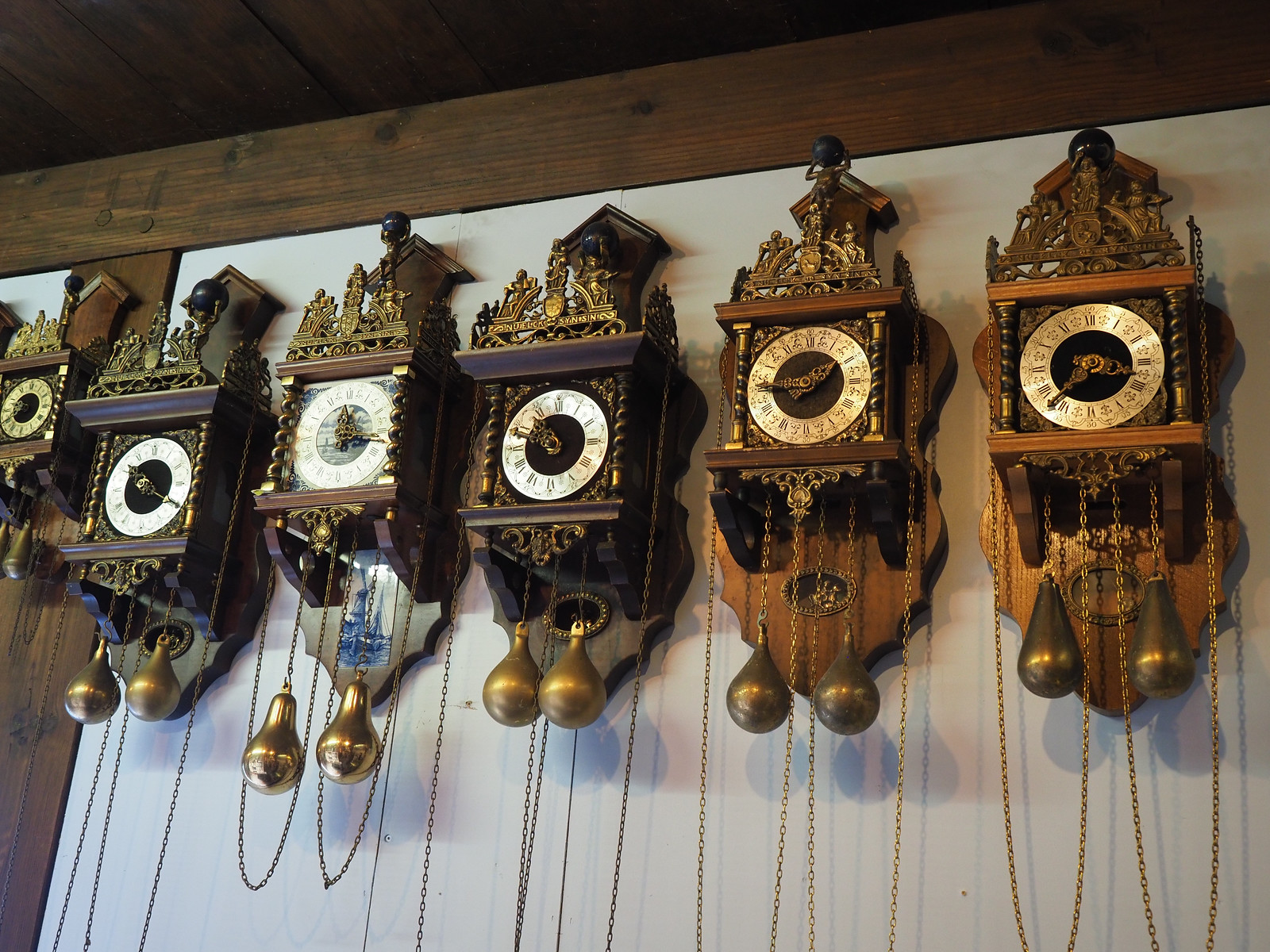This color photograph vividly captures a display of six ornate antique clocks, resembling a blend between grandfather and cuckoo clocks. They are mounted on a white wall with dark brown trim, some of which emphasizes their prominence. Each clock, crafted from woods of varying shades—from light to dark—features an intricate, square-shaped design. The clock faces are round and made of a shiny silver metal adorned with Roman numerals and golden hands. Above each face, a detailed golden carving depicts Atlas holding a dark-colored crystal ball, accompanied by other elaborate gilded designs involving people or possibly animals.

The clocks have distinctive dual teardrop-shaped pendulums hanging from them, crafted from brass with gold chains that extend downward, adding to the overall ornate appearance. At the bottom of each clock, additional wooden features complement the antique aesthetic. Notably, five of the clocks are clearly visible, while the one on the far left is partially obscured and appears smaller. The setup is completed by a wooden ceiling and a decorative wooden panel above the clocks, suggesting a setting that could be a store or a specialized display area, emphasizing their beauty and craftsmanship.